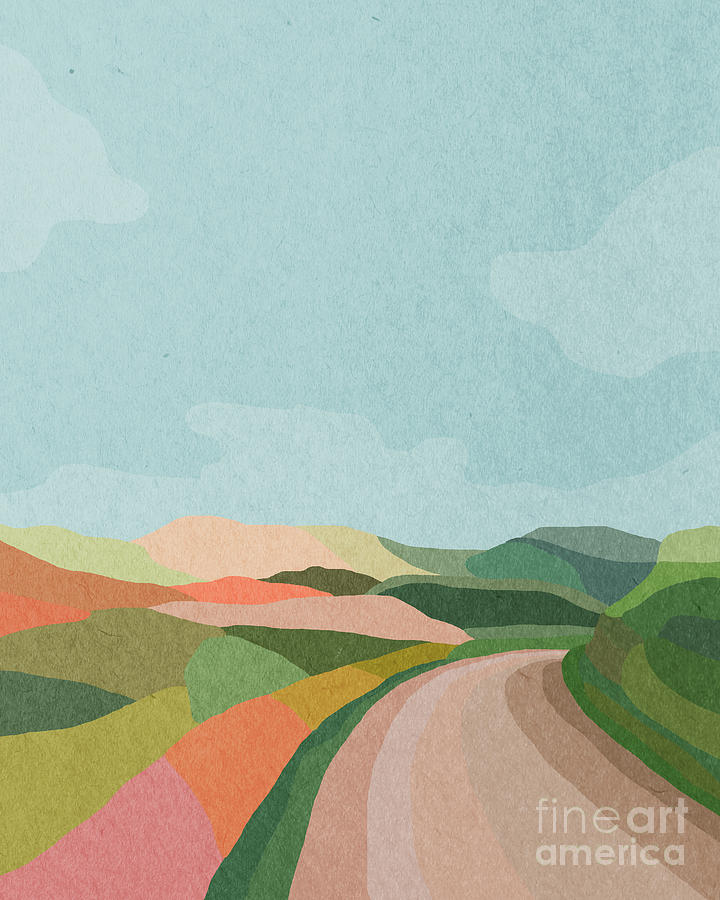The image is a vibrant, stylized painting titled "Fine Art America," indicated by the transparent white text in the bottom right corner. It portrays a winding dirt road that starts from the lower left and curves to the right middle portion of the scene. The road is depicted with thick, curved lines transitioning from darker tan to lighter hues, then back to darker tan as it extends to the right. Surrounding the road are various patchworks of simplistic shapes creating a natural landscape. On the right, there's an area of green grass formed by geometric shapes, resembling a green mountain. The left side features multicolored hills in shades of orange, green, peach, and brown. The sky above is composed of two flat, solid colors: a lighter blue with darker blue, suggesting clouds. The entire artwork is characterized by a collage-like style, where different shades are juxtaposed without blending, similar to pieces of cut-out cardboard paper assembled into a cohesive image.